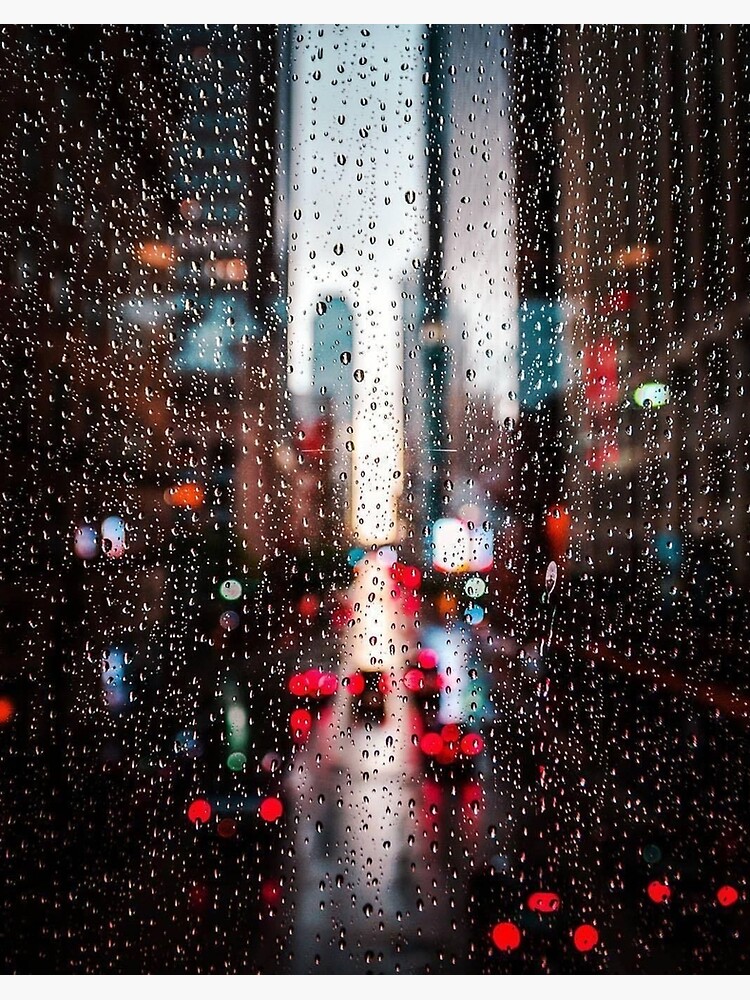The photograph captures a rainy scene through a window drenched in water droplets that create a beaded curtain effect. The focus is sharply on the raindrops, blurring the cityscape beyond. The city road cuts through the middle from the foreground to the background, bordered by skyscrapers on both sides. Prominent red brake lights of vehicles illuminate the wet road, adding splashes of color. Despite the daylight, the scene outside appears obscured by the rain and the blur, with indistinguishable buildings and a cacophony of red, blue, gray, purple, and white lights dotting the image. The overall effect is a vivid yet indistinct portrayal of a bustling, rainy city.